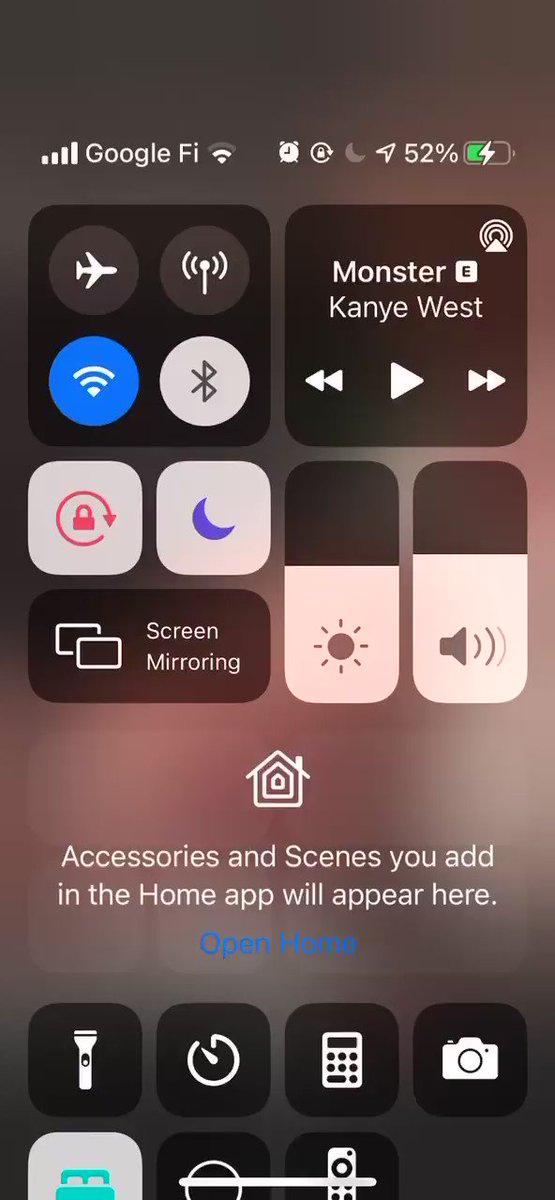Detailed Caption:

The image showcases a phone’s interface against a gray background. At the top, indicators for Google Fi service and an ongoing alarm are visible along with a battery icon showing 52% charging. Nearby, an airplane mode icon is displayed within a circle, signifying that airplane mode is enabled. 

The screen also includes a Wi-Fi signal indicator and a Bluetooth signal indicator, both enclosed in circles to show their active status. Additionally, there's a white square icon with a lock symbol encircled, likely representing a locked screen, and another white square icon featuring a blue moon, suggesting the 'Do Not Disturb' mode is on.

At the center of the display, media controls are present with a play button flanked by rewind and fast-forward buttons, labeled "Monster Kanye West," indicating the song currently playing. Below that, two rectangular sliders are shown: one with a sunshine icon, representing screen brightness, which is slightly over halfway filled; the other slider also over half-filled representing speaker volume.

Further down, there's an icon for screen mirroring beside an image of a house with a caption reading, "Accessories and scenes you add in the home app will appear here." This section is accompanied by a blue "Open Home" link.

Finally, at the bottom of the screen, there are seven small square icons, possibly representing various applications or shortcuts, neatly aligned at the bottom.